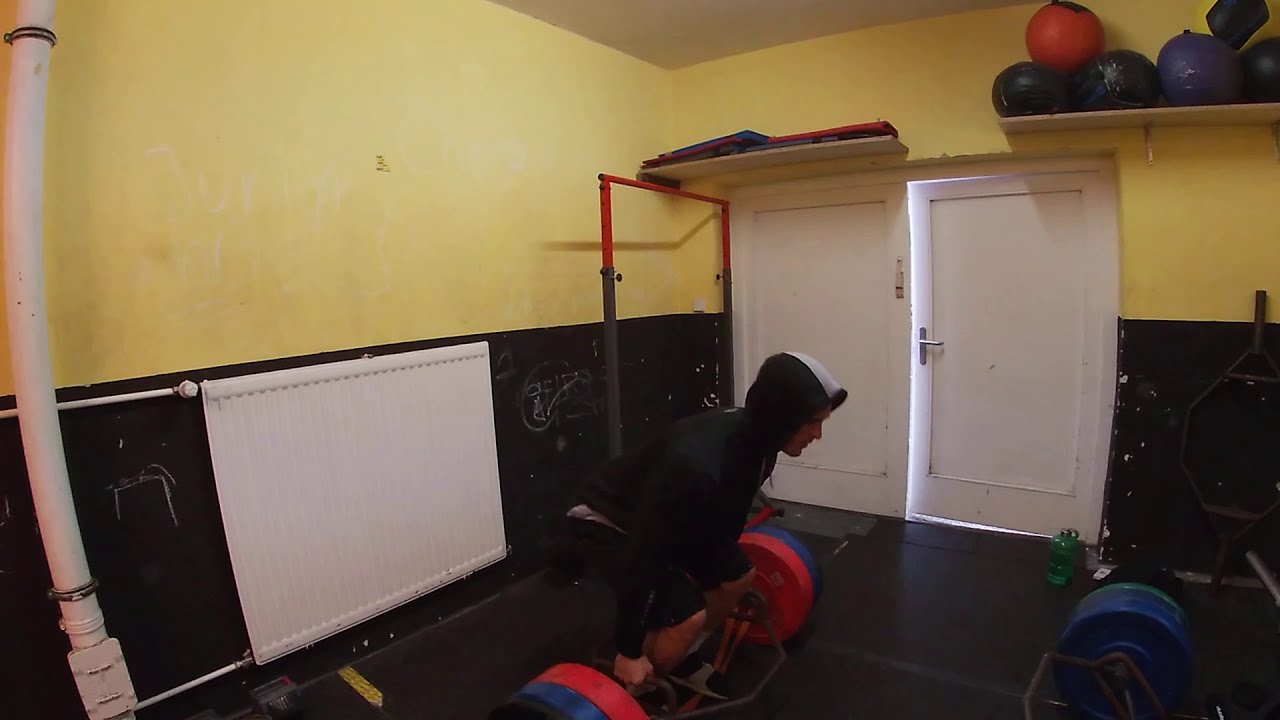In an indoor room that appears to be a home gym, a young man is captured in the middle of a weightlifting exercise. The room features two white doors with a cracked open allowing some light to spill in. The upper part of the wall is painted yellow, while the bottom part is black, creating a distinct separation. On the left side, a white heater is mounted against the black section of the wall. 

Centrally featured in the image, the man is squatting, preparing to lift a barbell with blue, red, and black weights attached. He is dressed in a black and white hoodie with the hood up, and black shorts. Several deadlift bars are present, including one in front of him with weights stacked on it and another propped against the wall. 

Above the two white doors is a shelf holding several medicine balls, and there are additional mats on another shelf to the right. A few scattered items, including a water bottle, a cell phone, and a gym bag, lie on the floor nearby, presumably belonging to the man. The floor has a rubber gym surface, complementing the functional yet minimalist setup of this home workout space.